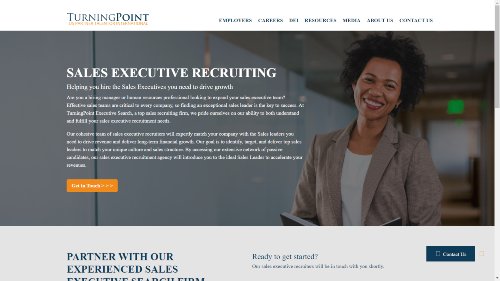The website titled "Turning Point" appears to specialize in sales executive recruiting. The homepage features a stock photo—or possibly an authentic one—of a light-skinned Black woman smiling in an open office environment. The top navigation menu includes links such as "Employers," "Careers," "Contact Us," and "About Us." Below the main banner image, a prominent message reads "Partner with our experienced sales executive search team," followed by a "Ready to get started" prompt. The overall design is functional with a light gray theme that continues as you scroll down. There's also a small, unclear tagline beneath the Turning Point logo.